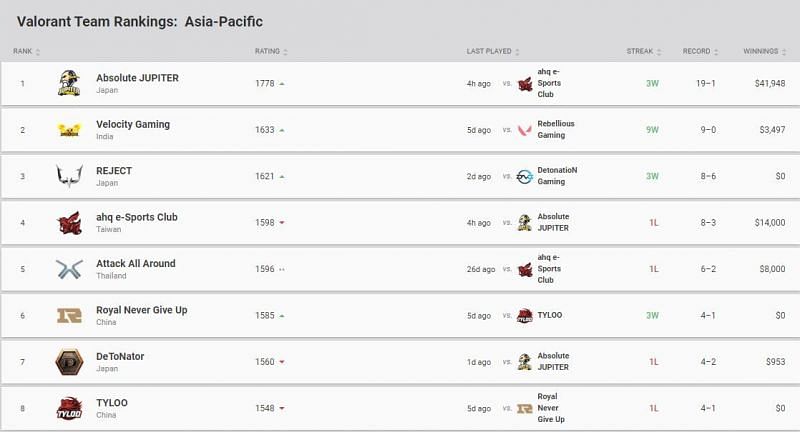A computer screen displays the "Valorant Team Rankings: Asia-Pacific" in a spreadsheet format consisting of rows and columns. The rankings span from 1 to 8, starting with 1 at the top and 8 at the bottom left-hand corner. The teams listed are:

1. Absolute Jupiter (Japan)
2. Velocity Gaming (India)
3. Reject Japan (Japan)
4. Esports Club Taiwan (Taiwan)
5. Attack All Around (Thailand)
6. Royal Never Give Up (China)
7. D-Detonator (Japan)
8. Tai Lu (China)

Each team is rated with numerical values in the thousands, aligned in the "Rating" column. The "Last Played" column indicates the time since each team's last game, listed either in hours or days. Additional sections display each team's "Esports Club," "Streak," "Record," and "Winnings," summarizing their recent performance and monetary earnings.